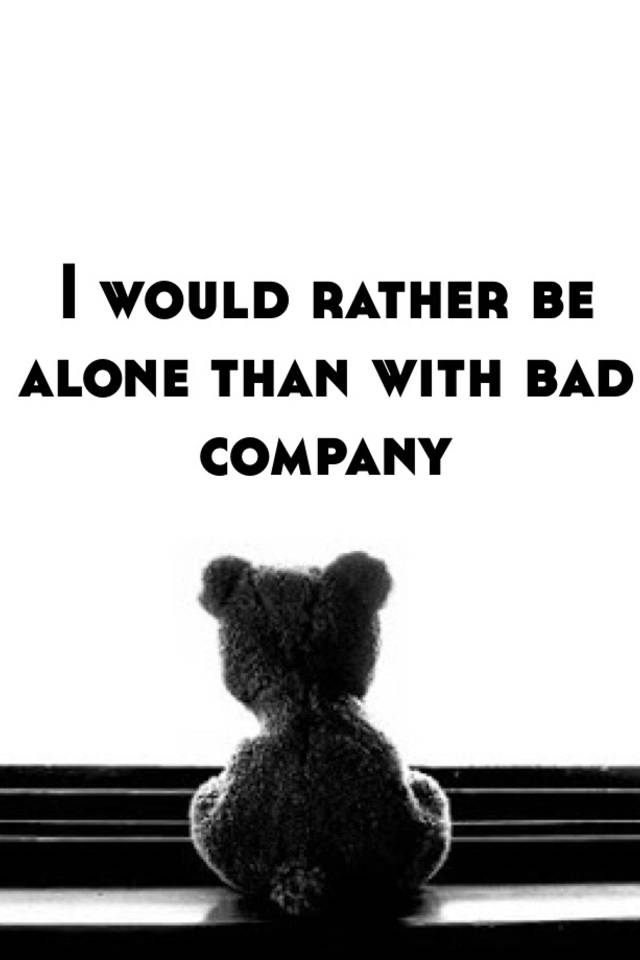In this evocative black-and-white photograph, the somber back view of a teddy bear is captured as it sits upright, gazing out a window. The only visible details of the teddy bear suggest it is brown in color, although the washed-out monochrome tones conceal its specifics. Bold, capitalized black text above the bear poignantly reads, "I would rather be alone than with bad company." The window frame, with its distinct grooves, comes up to the teddy bear's leg, and the bear sits pensively on a light-colored wooden platform or ledge. A slight shadow casts beneath it, adding to the melancholic ambiance. The image has a vertical rectangular format, reminiscent of an internet meme, capturing a lonely yet introspective indoor scene.